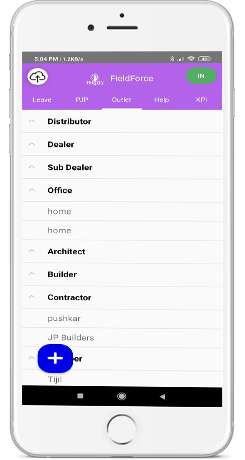A white smartphone with a white bezel is prominently featured in the image. The device displays a large round button centered on the bottom bezel. At the top bezel, a microphone and possibly a front-facing camera are visible. The screen shows a "Field Force" page, characterized by a purple banner at the top, indicating it is a cloud service utility. A small icon featuring a black and white cloud with an upward-pointing arrow is situated on the left side, suggesting the app is used for cloud uploads. Below the banner, several entry field options are listed, including "Distributor," "Dealer," "Sub-dealer," "Office," "Architect," "Builder," and "Contractor." Additionally, a prominent blue rounded button with a plus sign is superimposed along the bottom of the screen. Beneath this, a black ribbon banner displays the three primary smartphone control icons.